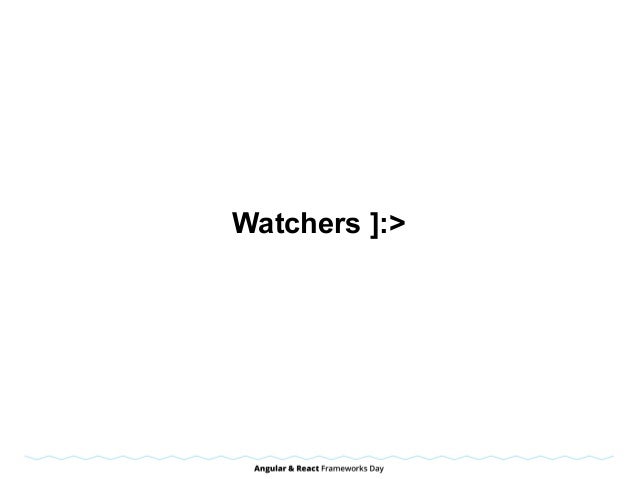The image has a stark white background with centrally positioned text. In plain black font, the word "WATCHERS" stands prominently, with all letters capitalized. To the right of this text, there's a text emoji constructed from a bracket, a semicolon, and a sideways caret, resembling a happy face. Near the bottom of the image, a wavy, light blue line spans the width of the image horizontally. Beneath this line, in very small, dark text, it reads "Angular and React Frameworks Day."